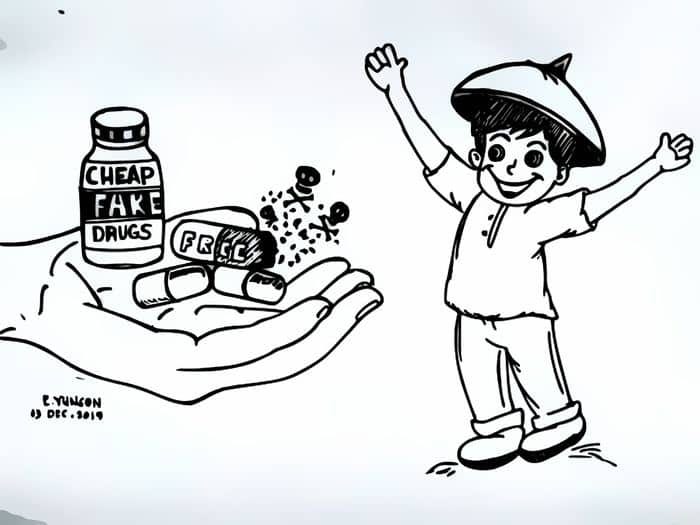In this black and white pen drawing, a young, happy Asian boy is depicted on the right side, with both arms raised in celebration and a wide smile on his face. He is wearing clothing along with a distinctive, perhaps traditional, hat. On the left side of the illustration, a hand is prominently featured, holding out several pills and a small medicine bottle labeled "cheap fake drugs." At least one of the pills is marked "free." Surrounding the hand and pills are danger symbols, including skull and crossbones, implying the harmful nature of these drugs. The background transitions from white in the middle to light gray at the top and bottom. Below the hand, the artist's name, Yungon, and the date, 13 December 2019, are inscribed, indicating when the drawing was created. The entire illustration starkly portrays the grave issue of children having access to dangerous, counterfeit medications.